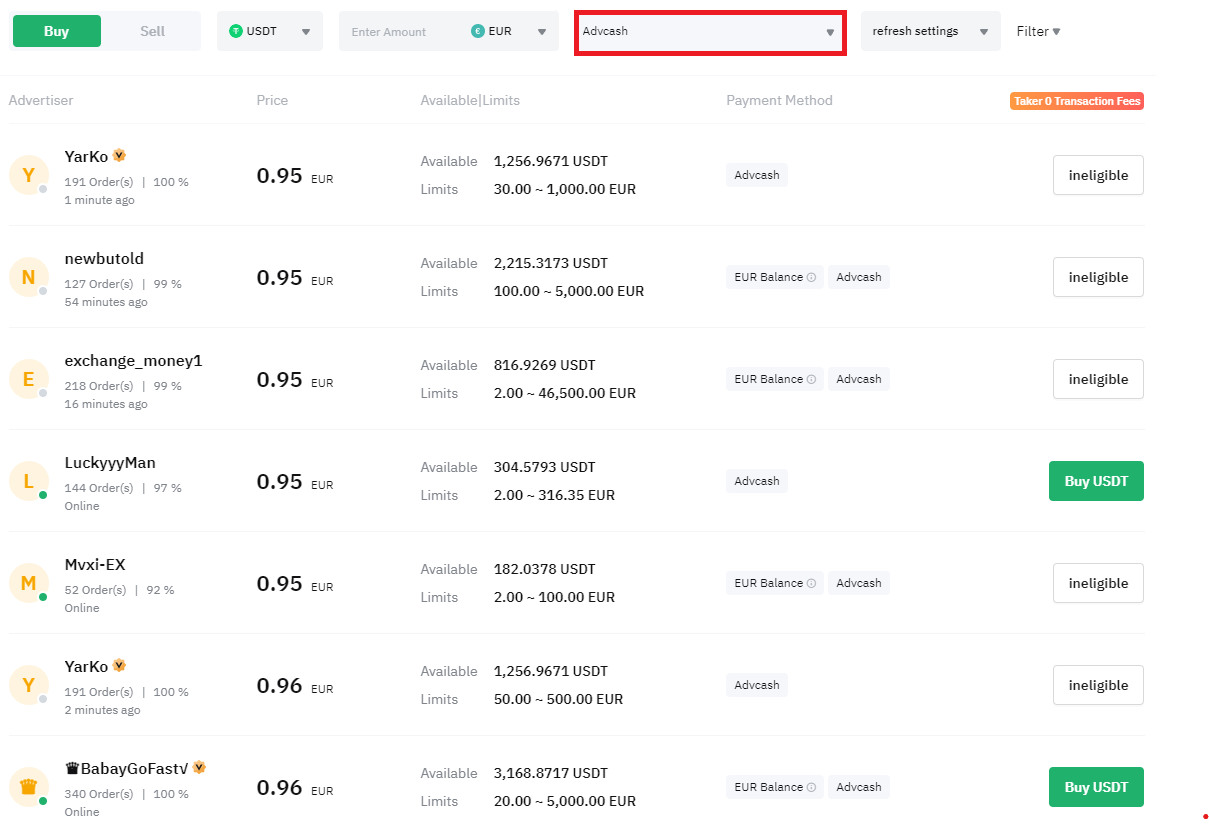This is a detailed screenshot of a trading application interface, potentially for trading stocks, cryptocurrencies, or currencies:

- **Top Section**: 
  - On the upper left corner, a green "Buy" button is prominently displayed, followed by a "Sell" option to its right.
  - The current trading pair shown is USDT (Tether) trading for Euros (EUR).
  - There is an option highlighted in a red rectangle, labeled "ADV Cash".
  - Additional settings such as "Refresh" and "Filter" features are available.

- **Main Table**:
  - The table comprises five columns labeled as: Advertiser, Price, Available/Limit, Payment Method, and Taker Transaction Fees.
  
- **Table Details**:
  - **Advertiser**:
    - "YARCO"
    - "new but told"
    - "exchange_money1"
    - "lucky man" (with three 'Ys')
    - "MVX1-EX"
    - "YARCO" again
    - "baby go fast"
  
  - **Price**:
    - Most listings show 0.95 Euros per USDT.
    - The latest entries by "YARCO" and "baby go fast" list the price as 0.96 Euros per USDT.
  
  - **Available/Limit**:
    - Availability ranges with "YARCO" showing 1,256.9671 USDT with limits of 30 to 1,000 Euros.
    - Other entries have similar structured information but with different specified quantities and limits.
  
  - **Payment Method**:
    - Various options like "ADV Cash" and "Euro Balance".
    - Repeated patterns are observed, with a mix of "ADV Cash" and "Euro Balance" for most entries.
  
  - **Taker Transaction Fees**:
    - Taker fees show "ineligible" for several entries, with some listings specifically noting "Buy USDT" as ineligible.

- **Footer**:
  - There is a substantial orange background noting "Taker Zero Transaction Fees".

This interface appears to detail a complex trading scenario with various sellers listing their USDT for Euro, each presenting their specific prices, available quantities, and accepted payment methods.